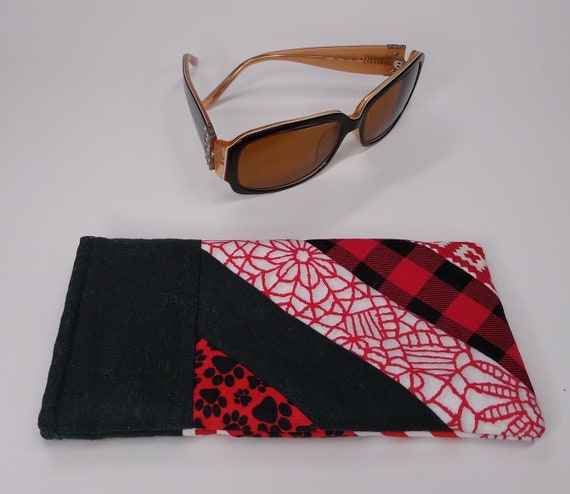In the image, a pair of sunglasses takes center stage against a predominantly gray background. The sunglasses have brown lenses with black frames, transitioning to dark brown and then light brown where they rest over the ears. The glasses cast a noticeable shadow on the surface. Below the sunglasses lies a folded cloth with a complex pattern. The cloth is predominantly black on the left side, transitioning to various strips featuring different designs: black paw prints—likely from a dog or cat—on a red background; a black stripe; red floral designs on a white background; a plaid stripe with checkered black, gray, and red lines; and additional red areas. In the top right corner of the cloth, there is a red plus sign within a red diamond shape, set against a white background.